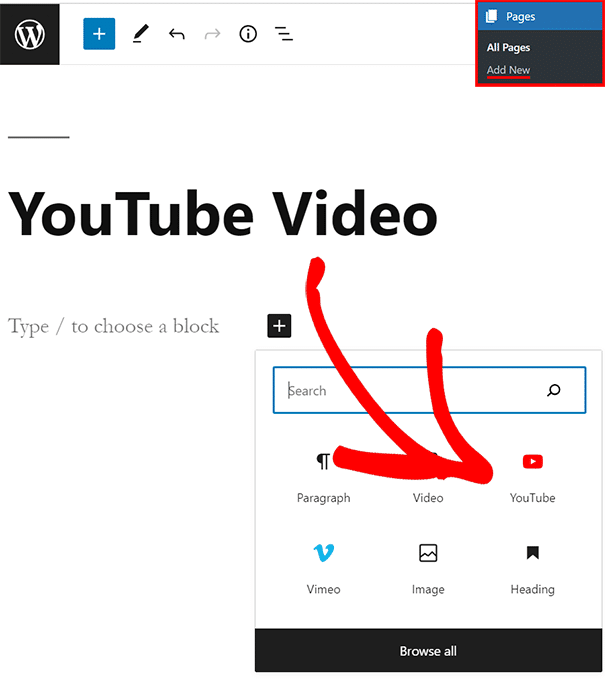The image features a webpage mockup with various elements highlighted for instructional purposes. At the top, there is a prominent banner, a headline, and a large, photoshopped red arrow pointing to a specific section of the site. 

In the upper left-hand corner, there is a black square with a white circle inside it, containing the letter "W". To the right of this on the white header, there are several icons: a blue square with a white plus sign indicating the add function, a pen marker signifying the edit function, undo and redo buttons for navigation, an information button depicted as an eye within a circle, and a three-lined icon for additional settings. 

In the upper-right corner, the words "Pages" in blue, "All Pages," and "Add New" are visible. Notably, the "Add New" button is underlined in red and enclosed in a red square to draw attention.

Below, on a white background, are the words "YouTube video, type slash to choose a block," with the red arrow pointing directly at the YouTube play icon. Additionally, a section with a search bar includes clickable options for "Paragraph," "Video," "YouTube," "Vimeo," "Image," "Heading," and "Browse All."

This detailed descriptive caption highlights each element and its function, providing a comprehensive overview of the image's content.